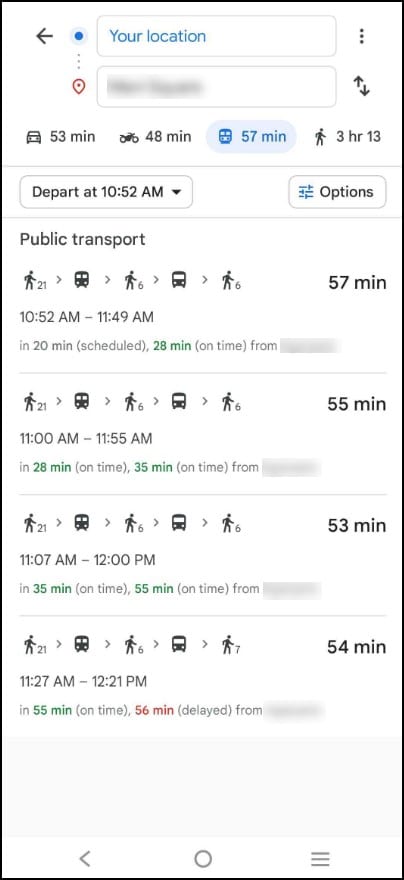An image depicting various transit options is highlighted by a blue dot that signifies the current location. The image details multiple transportation methods with corresponding travel times. By car, the journey is estimated to take 53 minutes; by bicycle, 48 minutes; and by bus, 57 minutes. Walking takes approximately 3 hours and 13 minutes. 

The departure time is set for 10:14 AM, and the slide illustrates various combinations of walking, bus rides, and transfer schedules. One specific route outlines a walking-bus-walking-bus sequence totaling 57 minutes, departing at 10:52 AM and arriving at 11:49 AM, with all segments on time ranging from 9 to 20 minutes each.

Another route requires a walking-bus-walking-bus combination totaling 55 minutes, from 11:00 AM to 11:55 AM, matching the previous on-time intervals. A third option shows a walking, bus, walking pattern separated by distinct times, amounting to 53 minutes, from 11:07 AM to 12:00 PM, with varying punctuality from 35 to 55 minutes.

Furthermore, a fourth route described includes walking (21 minutes), a bus ride, followed by a walking section (6 minutes), another bus ride, and concluding with a 7-minute walk, totaling 54 minutes, from 11:27 AM to 12:21 PM, experiencing 55 minutes on time and a delayed segment of 56 minutes.

Additional details are noted in the bottom left-hand corner of the image, where a hamburger menu icon is visible for more options.